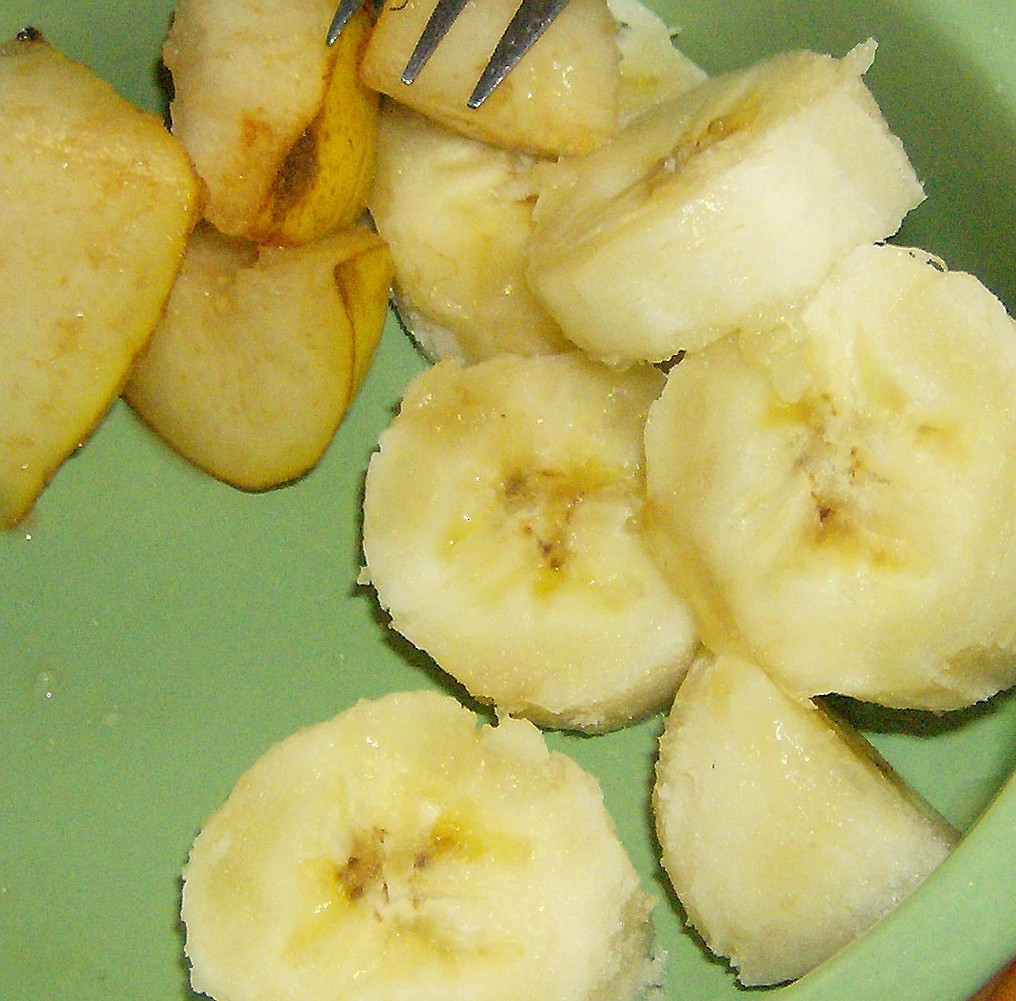This close-up photograph captures a bowl of sliced fruits arranged in a light green, plastic-looking bowl. Dominating the right side of the bowl are five circular slices of ripe banana, neatly positioned alongside what appears to be a quarter-cut banana slice tucked in the bottom right corner. Emerging from the top center of the image, the tips of a three-pronged fork are visible, poised perhaps to pick up the fruit. In the top left of the image, there are three or four slices of a different fruit, likely a pear still clad in its skin, adding a contrasting texture and color to the composition. The bottom left section of the bowl remains uninhabited by any fruit, showcasing a solid, calming green backdrop that emphasizes the fresh, vibrant appeal of the sliced fruits.